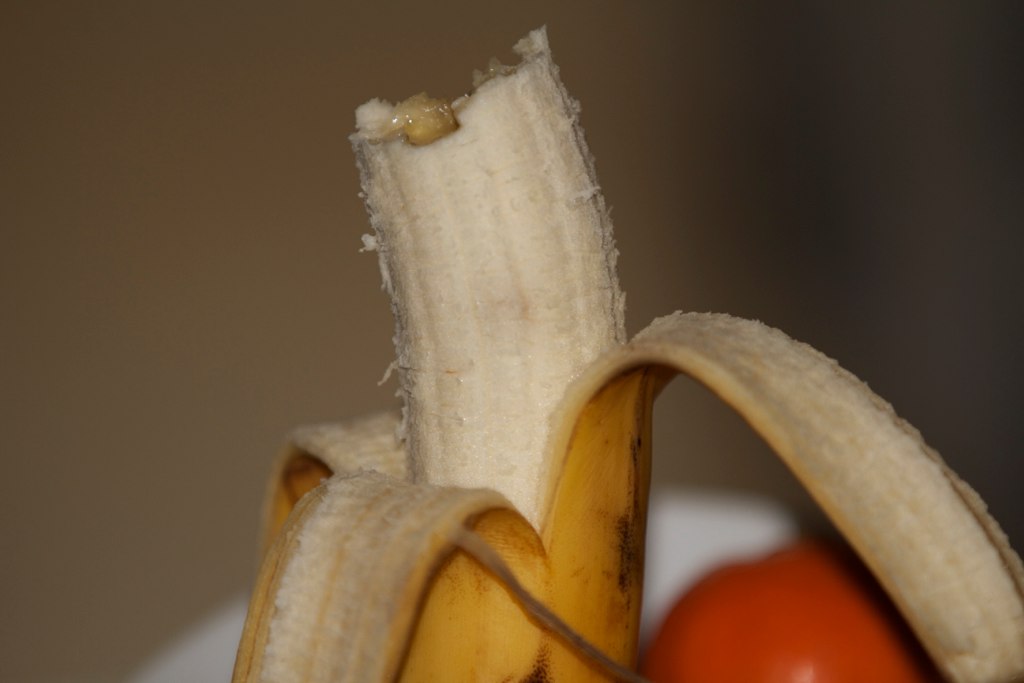This close-up photograph, taken indoors, beautifully captures a ripe banana in vivid detail. The camera's focus is sharply on the banana, leaving the background artistically blurred into an indistinct brownish hue. A hint of white and a splash of red or orange, possibly a piece of fruit or a tomato, add subtle color variations to the backdrop. The banana's golden-yellow skin, speckled with numerous brown spots and bruises, reflects its peak ripeness. The banana has been partially peeled, with three strips of skin hanging loosely around its middle, exposing the creamy white fruit within. The tip of the banana is missing, perhaps bitten off or torn away, revealing a flattened edge that suggests recent consumption.